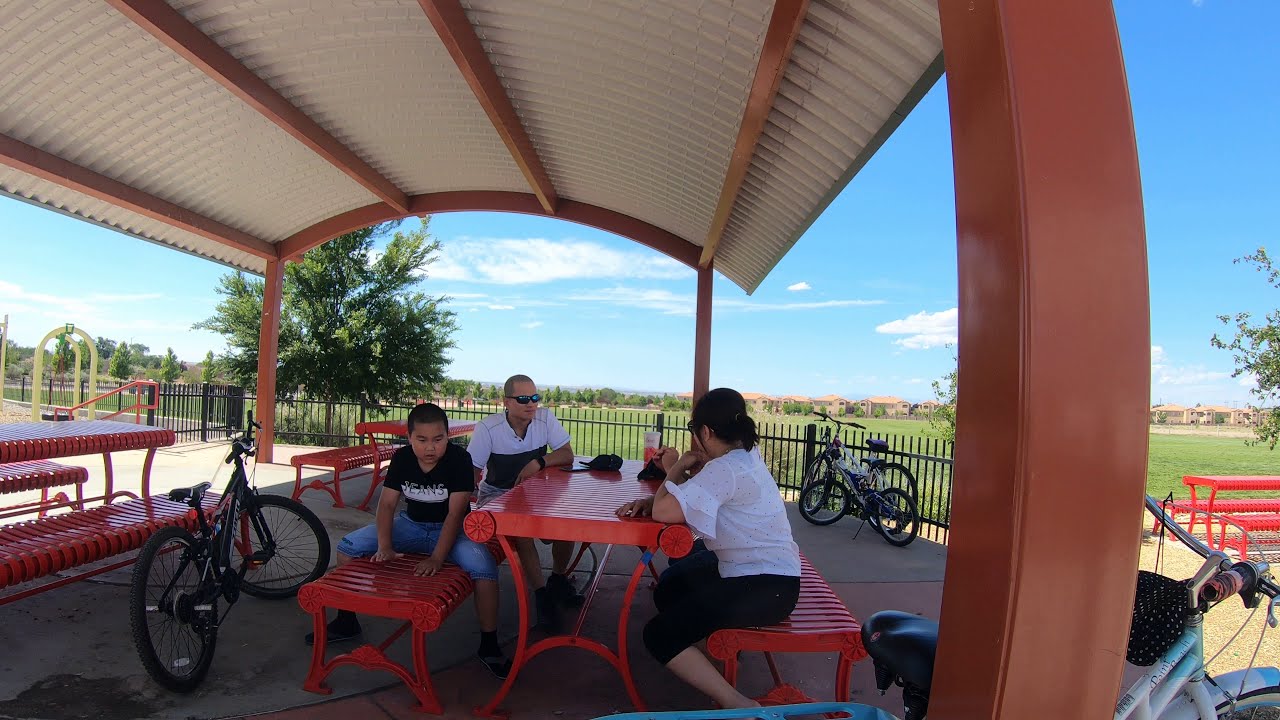This photograph captures an outdoor patio area bathed in sunlight, beneath a white-roofed and brown support-beamed pavilion that provides ample shade. Against a backdrop of light blue sky adorned with wispy white clouds, you can see several multi-story apartment buildings in the distance. The pavilion is set in a large, grassy field that stretches towards the horizon.

In the foreground of the image, the cement-floored patio boasts multiple metal-slotted tables and chairs. At the front-most table under the pavilion, four individuals are seated. A young boy, straddling a bench and facing the camera, wears a dark t-shirt with blue jean shorts. Across from him sits a woman dressed in a white shirt and dark pants, her back to the camera. Beside them, a man, wearing a white and dark t-shirt with glasses, faces the woman, engaging in conversation.

Surrounding the pavilion area, various bicycles are propped up against a black fence that partially encloses this space. Adjacent to the patio, there are additional red tables and benches, and a sandy or dirt area separates the pavilion from the expansive green field. Overall, this picturesque scene of a sunny day reflects a serene and communal atmosphere within an inviting park setting.